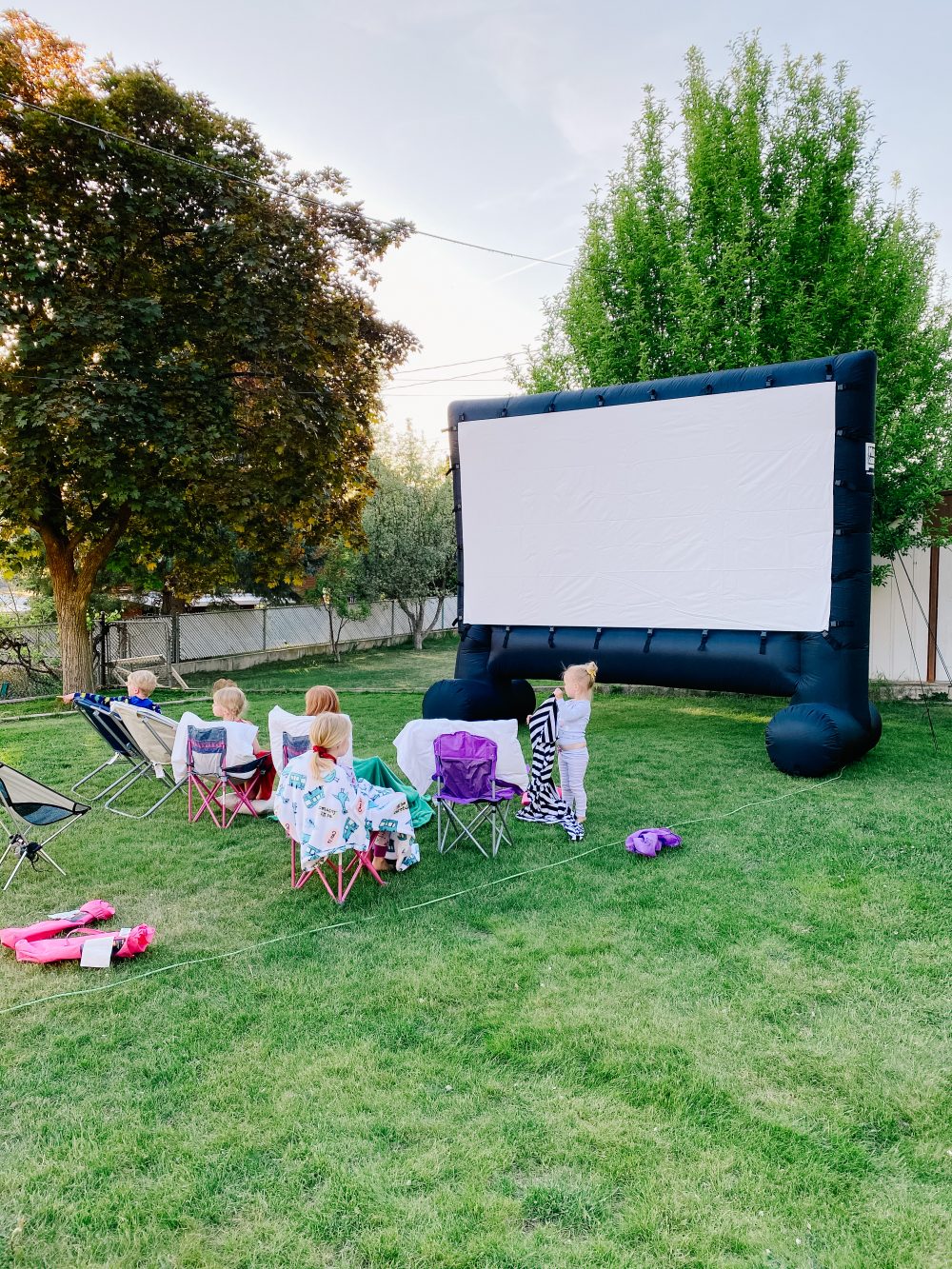In this vibrant daytime image, a group of young children, mostly with blonde hair, eagerly awaits an outdoor movie in a lush backyard. The scene is illuminated by a clear blue sky and framed by tall green trees, hinting at late summer with a few leaves starting to turn yellow. The expansive green lawn is enclosed by a white vinyl fence, providing a safe, cozy environment.

Dominating the upper right-hand corner is a gigantic blue inflatable movie screen with dark blue horizontal cylinders at its base and a white front where the movie will be projected. This screen shows subtle ripples, likely from being folded up before setup. In front, at least six children, dressed in their pajamas and wrapped in blankets, are seated in a variety of colorful lawn chairs. The padded chairs add a splash of color to the green backdrop. Despite it still being daylight, the children are all turned to their left, perhaps anticipating the start of the film or looking for someone to begin the show. The scene captures a perfect blend of anticipation and youthful innocence, ready for a magical evening under the open sky.